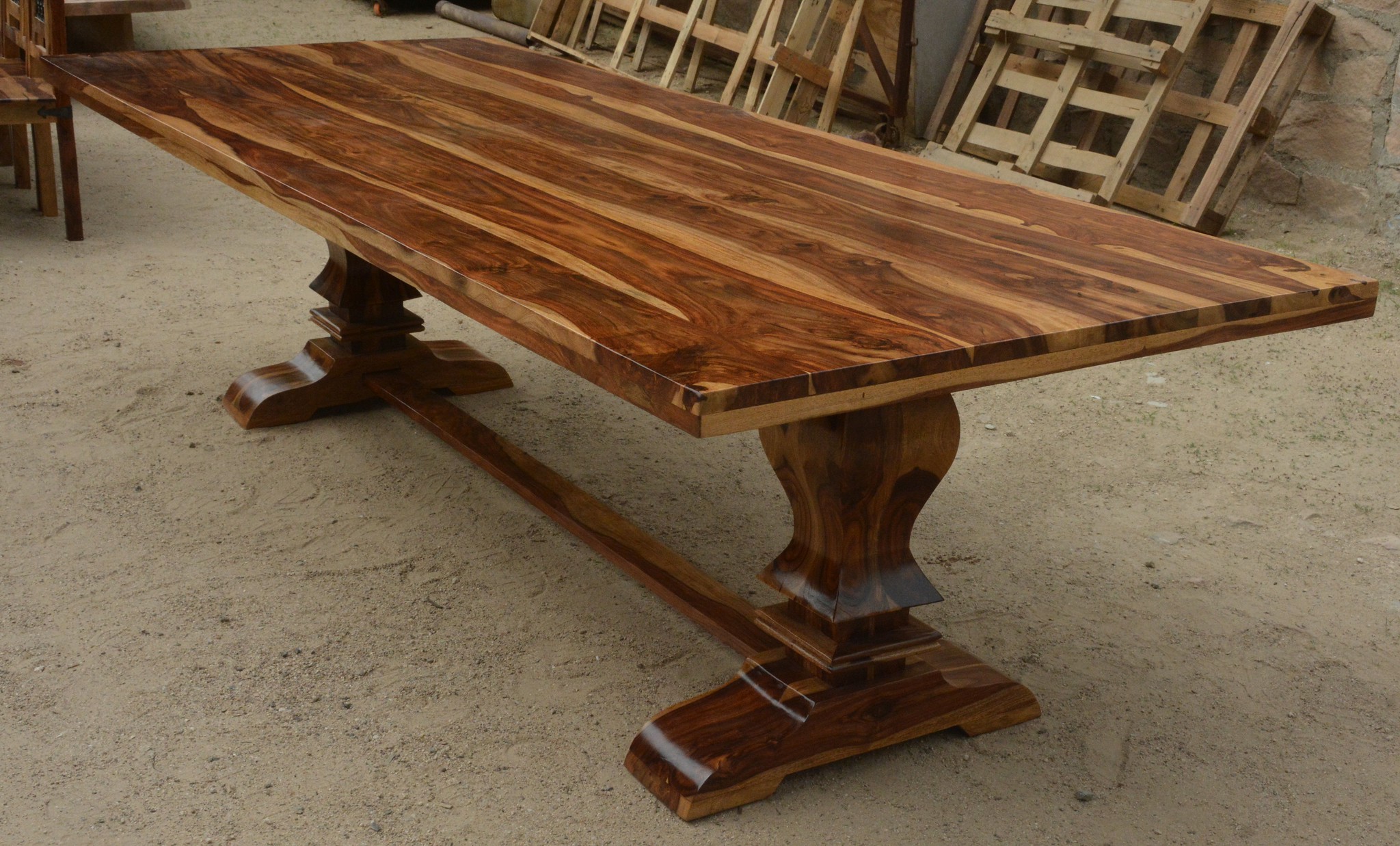This close-up photograph features a central wooden table, showcasing its robust, polished design with a shiny lacquer finish on both the tabletop and the legs. The table is crafted from thick wood with prominent beige grain patterns, resembling a mahogany hue, giving it a refined yet rustic appeal. The legs of the table are somewhat short, leading down to a lower square support and finally to long rectangular feet, also polished with lacquer. A connecting brown beam runs between the legs, adding stability.

The setting appears to be a garage or workshop with a dirt floor, complemented by a light brown, stone-like wall in the background. Surrounding the table are several elements of interest: a slice of a wooden dining chair with two visible legs in the upper left corner, suggesting a similar style to the table, and additional wooden palettes and scaffolding resting against the wall. These palettes, along with other unfinished wooden pieces, hint at ongoing woodwork projects. Another wooden table can be seen peeking out from behind the chair, reinforcing the workspace atmosphere.